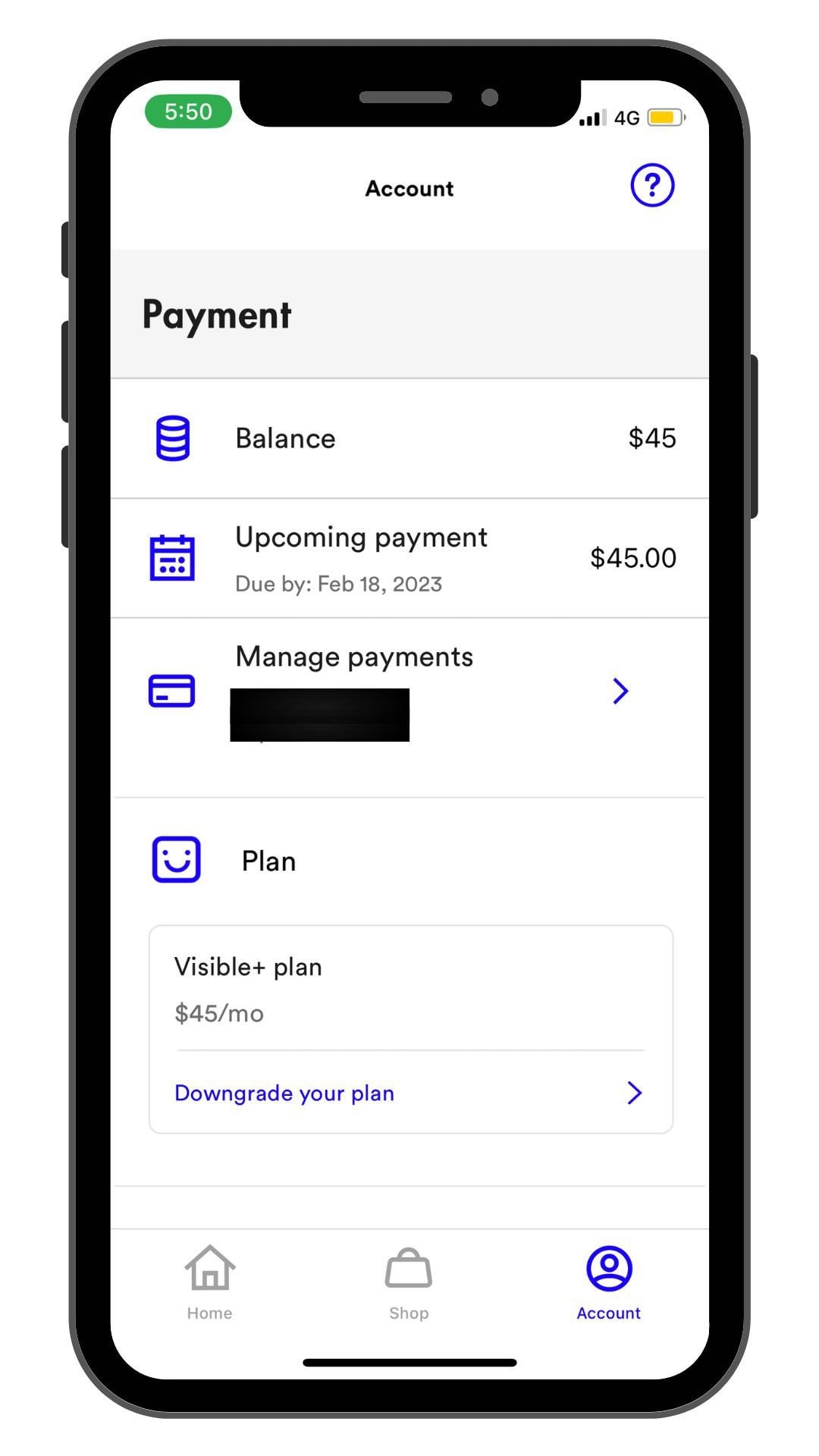The image displays a smartphone screen with a multitude of details regarding account information. At the top of the screen, a black border frames the display. In the upper left corner, there is a green box displaying the number "550." Next to this, the signal strength indicator shows three out of four bars, signifying a 4G connection. Additionally, the battery icon indicates approximately 80% charge.

Below this status bar, the screen shows a section labeled "Account" with a blue-bordered circle containing a question mark in the center. Beneath this, there's a gray box with the word "Payment." 

Continuing downward, the background turns white and displays the word "Balance" along with an amount of "$45.00." A gray horizontal line separates this section from the next, which details an "Upcoming Payment" of $45.00, due by February 18, 2023. Following this, the words "Manage Payment" are visible alongside a black box partially obscuring some text, with a right-facing arrow (>) next to it.

Further down, the section is labeled "Plan" followed by another line break. It then reads "Visible Plus Plan $45.00 a month," with yet another line break beneath it. Finally, the option to "Downgrade Your Plan" is presented. The bottom of the screen features navigation buttons labeled "Home," "Shop," and "Account."